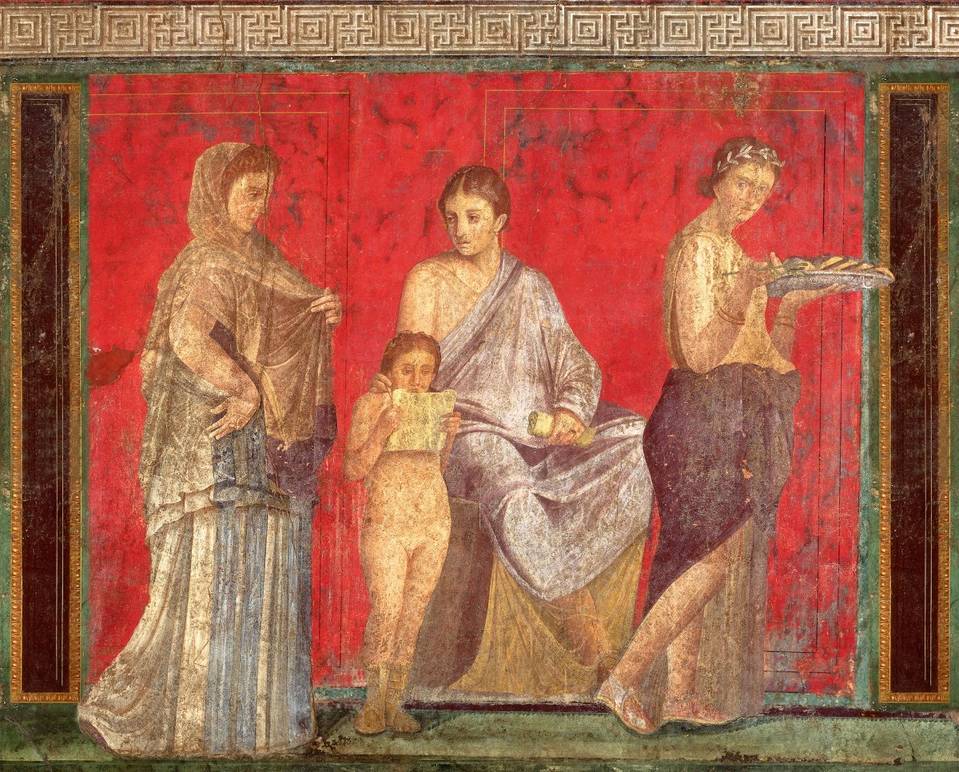The image is a detailed color photograph of a Roman fresco occupying the entire frame in a landscape orientation. At its center, a young man dressed in a white toga sits on a square cloth-covered chair and appears to be reading or holding a scroll. To his left, a young child, likely a girl with long hair, stands and reads from a piece of paper. On the far left side, a woman with reddish-brown hair wearing a long white skirt with gold brocade and a gold headscarf, which she holds in a graceful pose, looks down thoughtfully. To the right of the seated man, another female figure walks toward the right while facing forward; she is carrying a tray of food—possibly bread—and wears a long purplish skirt with a sheer gold layer underneath. Behind the figures, the background is vividly red with a hand-painted appearance, accented by a green marbleized border and a Grecian key motif band at the top. On either side of the fresco, there are dark burgundy marble vertical columns with gold trim. The overall style is a highly realistic portrayal, embodying photographic representationalism with the wear signs of an ancient mural, such as peeling paint and scratches, contributing to its historical ambiance.